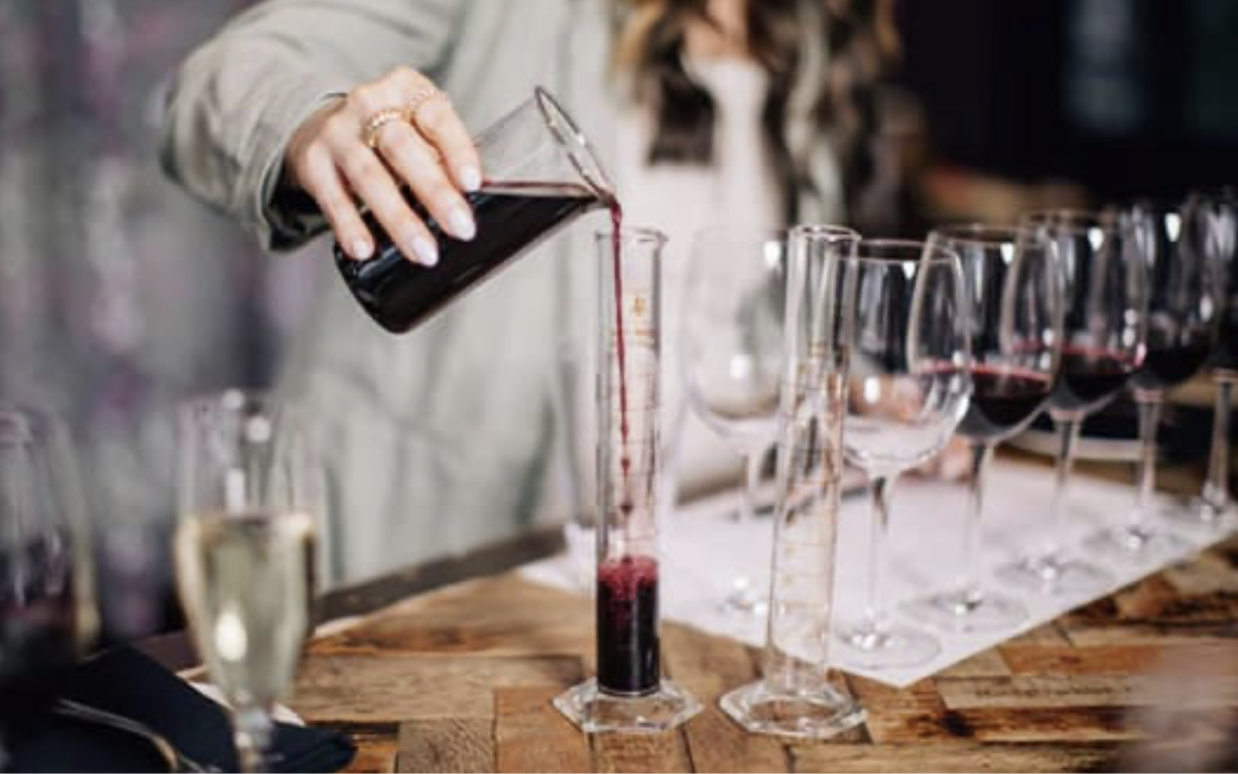The image depicts a close-up indoor scene of a wine-tasting party. The focus is on a woman with dark wavy hair and white skin, whose body is visible from the shoulders to the hips. She is adorned with rings on her fingers and has white nail polish. She is wearing a light green jacket. The woman is pouring a dark purple, burgundy wine from a glass beaker into a graduated cylinder using a long instrument. On the table in front of her, which has a wooden surface and a placemat, there are several wine bottles and a variety of wine glasses. Some of these glasses are empty, while others are partially filled with the burgundy wine. Additionally, there is a single glass of white wine located in the bottom left-hand corner of the image. A white piece of paper is also present on the table, contributing to the organized setting. The scene signifies an environment of measuring and equalizing wine servings, possibly for a tasting or blending event.